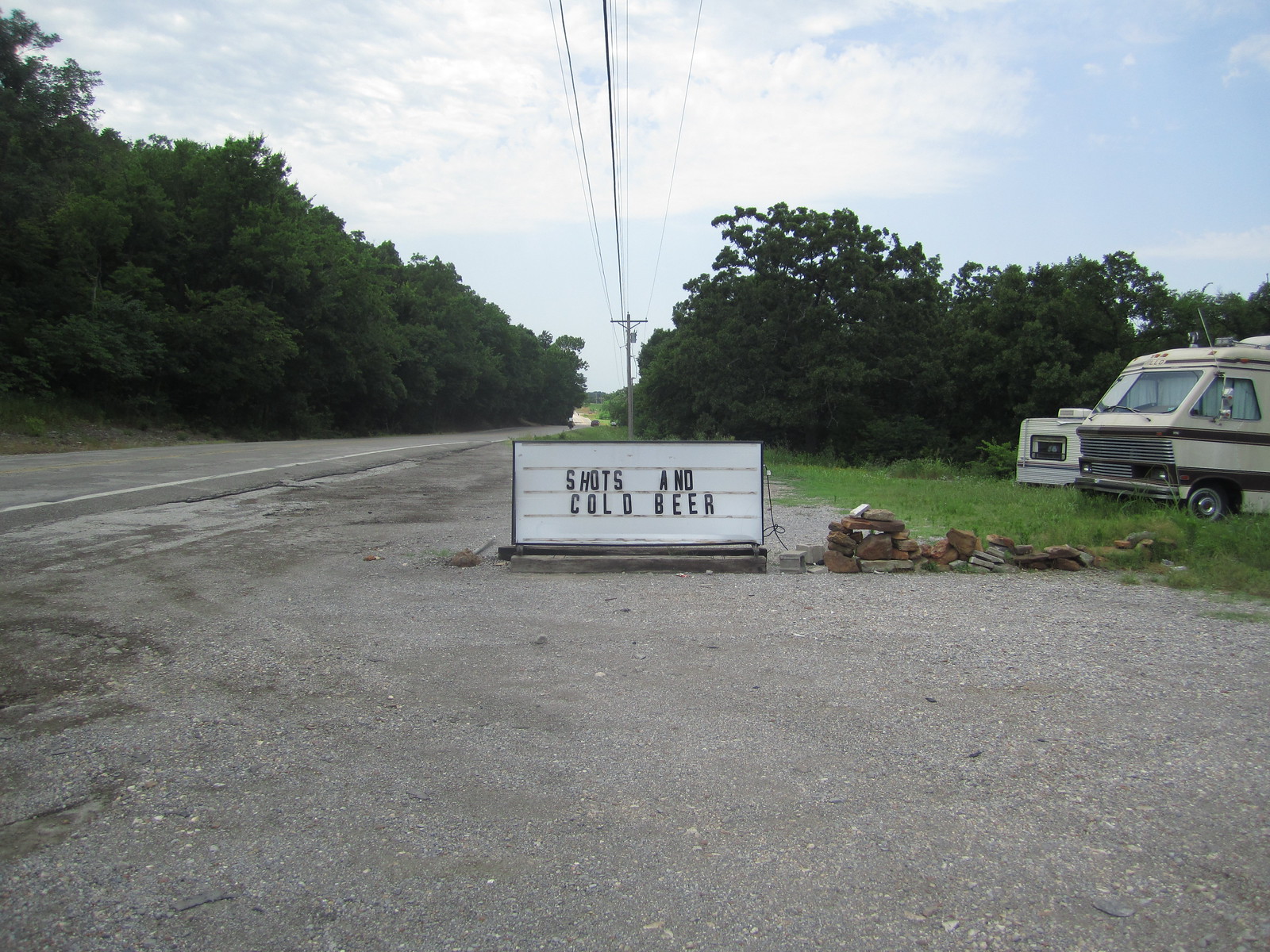Under a vibrant blue sky dotted with fluffy white clouds, a scene unfolds with utility poles and electric lines stretching into the distance. Flanking both sides of the image, verdant green foliage and leafy trees frame the view, interspersed with various patches of green vegetation. On the right side of the frame, a parked RV stands out against the predominantly gravel-covered ground, which shades a muted gray. A large road cuts through the middle of the scene, directing attention to a white sign that prominently advertises "Shots and Cold Beer." Just beneath this sign, a neatly stacked pile of wooden logs adds a rustic touch to the otherwise lively landscape.